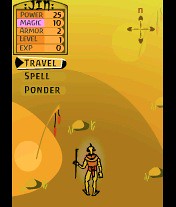This screenshot captures a nostalgic scene from an old-school video game, reminiscent of classic RPGs. The image, roughly passport photo-sized, features a character dressed in Egyptian attire walking down a desert path, vividly evoking the ambiance of ancient Egypt. At the top of the screen, the title "JIN" is displayed, possibly indicating the game's name. The gameplay interface includes a status bar on the top left, showing vital statistics: Power at 25, Magic at 10, Armor at 2, Level 1, and EXP at 0. Below this are options labeled Travel, Spell, and Ponder, hinting at the interactive elements of the game. On the top right, a compass indicates the character's orientation, with North clearly marked. The detailed interface and atmospheric setting suggest a richly immersive gaming experience, characteristic of the retro era.